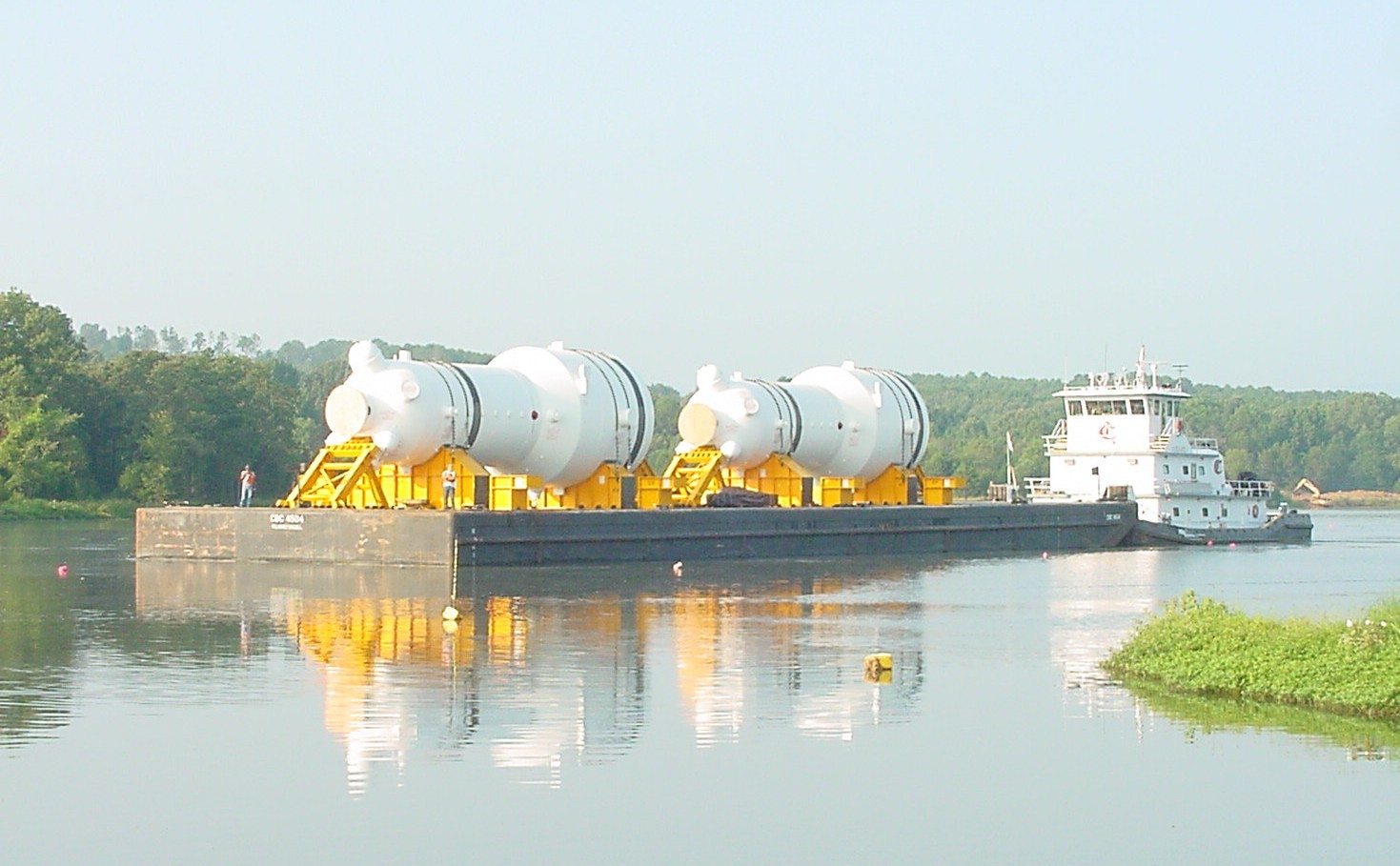The photograph captures a vibrant scene set along a waterway on a clear but slightly hazy day with a blue sky. Dominating the image is a tugboat pushing a barge upstream. The barge is laden with two enormous cylindrical white generators, lying on their sides, with one end larger than the other. These generators, snugly secured with plywood, planking, struts, and steel cables, are positioned atop yellow racks, highlighting the extensive measures taken to ensure their safe transport. 

In the foreground, a substantial buoy marks a turn in the river, while further up the waterway, a cement dock extends from the grassy knoll on the right side of the image. On this dock, standing on a brown wooden platform, are two gentlemen positioned near the corners, overlooking the transfer. Adjoining the platform is a large white boat with multiple windows, steps, and a visible flag post that is reflected in the water. This picturesque setting is framed by a dense tree line in the background, emphasizing the serene yet industrious nature of the scene.